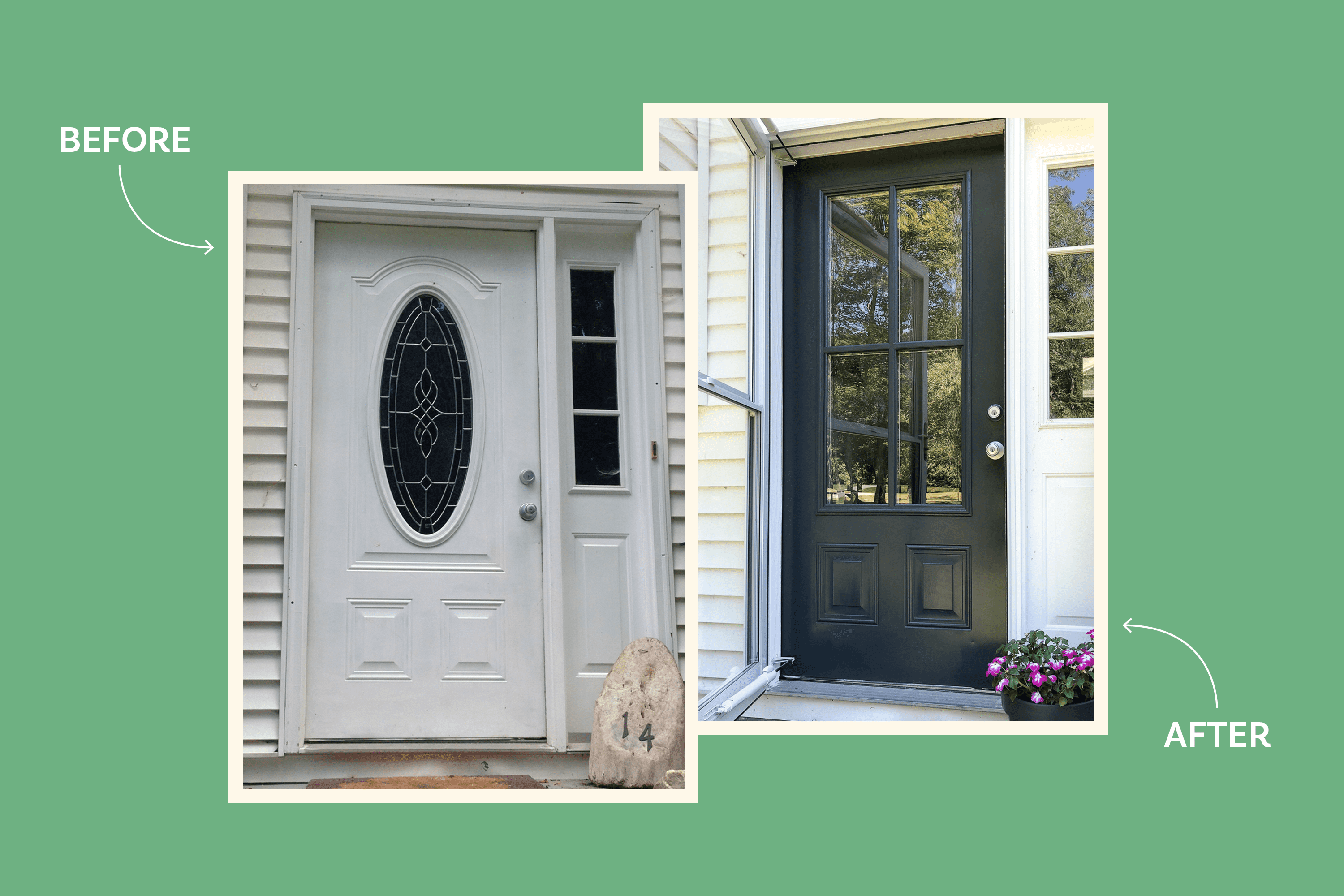This advertisement showcases a door replacement company and features a "before" and "after" image of a front door. The house in the image has white siding and a three-paneled vertical window adjacent to the front door on the right. 

The "before" image displays a white paneled door adorned with an oval-shaped stained glass section in the center, featuring diamonds and Celtic knots. There is also a brown doormat and a rock labeled with the number "14" in front of the door.

The "after" image presents a black paneled door with a significantly larger window section comprised of four panels, occupying the upper half of the door. Additionally, a two-paneled screen door is now installed, offering an option for increased light entry and modern appeal.

Both images are positioned diagonally against a pale green background, emphasizing the improved aesthetics and functionality after the door replacement. This visual comparison is ideal for those considering an upgrade to allow more light into their home or to modernize its appearance.